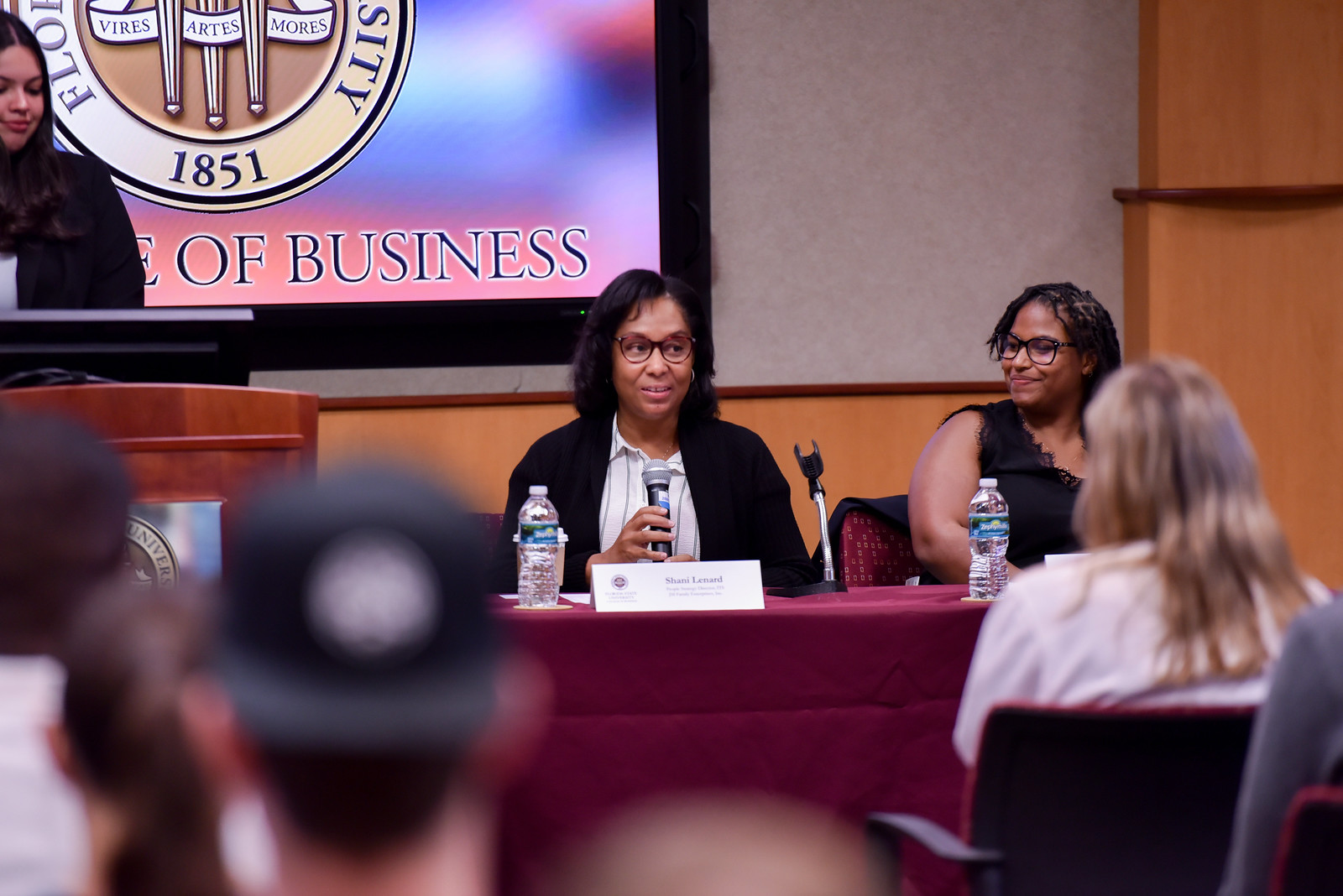In the image, a professional event or classroom setting, likely at a university, is depicted. At the upper left, a woman with dark hair and wearing a dark jacket stands at a podium with a lit screen behind her displaying partial text: "1851 of business" and "Veris Artis Moris." Below her, two African-American women are seated at a maroon-covered table connected to the podium. The woman in the center, wearing glasses, a black blazer over a white shirt with black stripes, is holding a microphone. Her name tag reads "Shani Leonard," and she has a cup of coffee and a bottle of water beside her. The woman next to her, also wearing black and glasses, has short medium black hair and is smiling at Shani. In the foreground, the audience includes a young blonde girl in a white shirt and a boy wearing a ball cap, seen from the back. The walls of the room are gray with wood panels, contributing to a formal and academic atmosphere. The image conveys a sense of engaged discussion or presentation in a university environment.